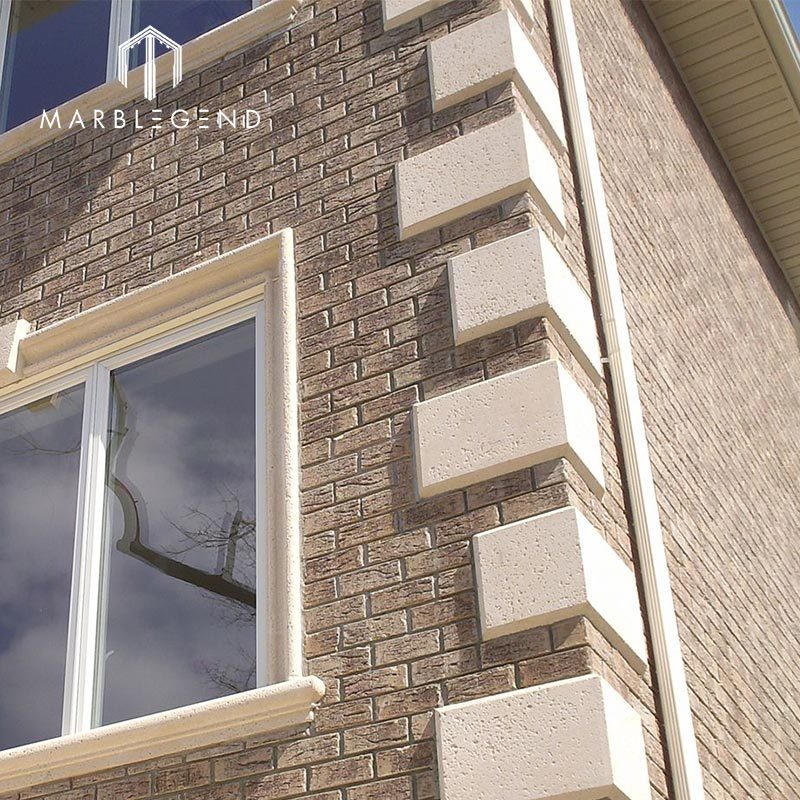The photograph features a corner view of a large brick building with soft beige and sandstone bricks. The structure prominently displays larger, white accent bricks on the corners, creating an offset pattern where they skip two of the smaller bricks below. The building's architectural details include a drainage pipe descending from the roof, visible on the right side. 

Two windows with white trim are present in the image. The lower window reflects the image of bare tree branches, adding a natural element to the scene. The sliding windows are on the left side of the building, contributing to the intricate brickwork.

Additionally, the top left corner of the image showcases a logo with the text "Marble Legend." The logo design mimics the corner of a building, where the E's are stylized with three horizontal lines stacked atop each other, providing a unique visual element. The photograph likely serves an architectural or real estate purpose, highlighting the building's structure and design elements in detail.